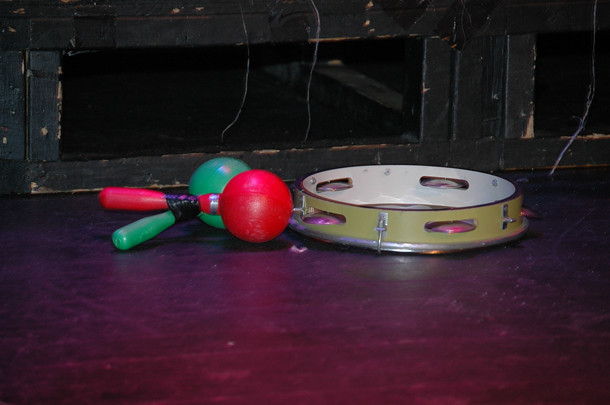The photograph captures a purplish-tinted wooden floor, suggesting a stage with colored lights reflecting off its surface. The background is comprised of used black wood with small square openings, potentially under-stage storage. Centrally placed on the floor is a tambourine, positioned face-down, indicating that the striking surface is against the floor. The tambourine is rimmed in yellow with silver metal cutouts along the sides and a white surface inside. To the left of the tambourine are two plastic maracas, one red and one light aqua green, taped together in an X shape. Additional stage equipment or a table with wires can be seen in the background, emphasizing the musical setup of the scene.